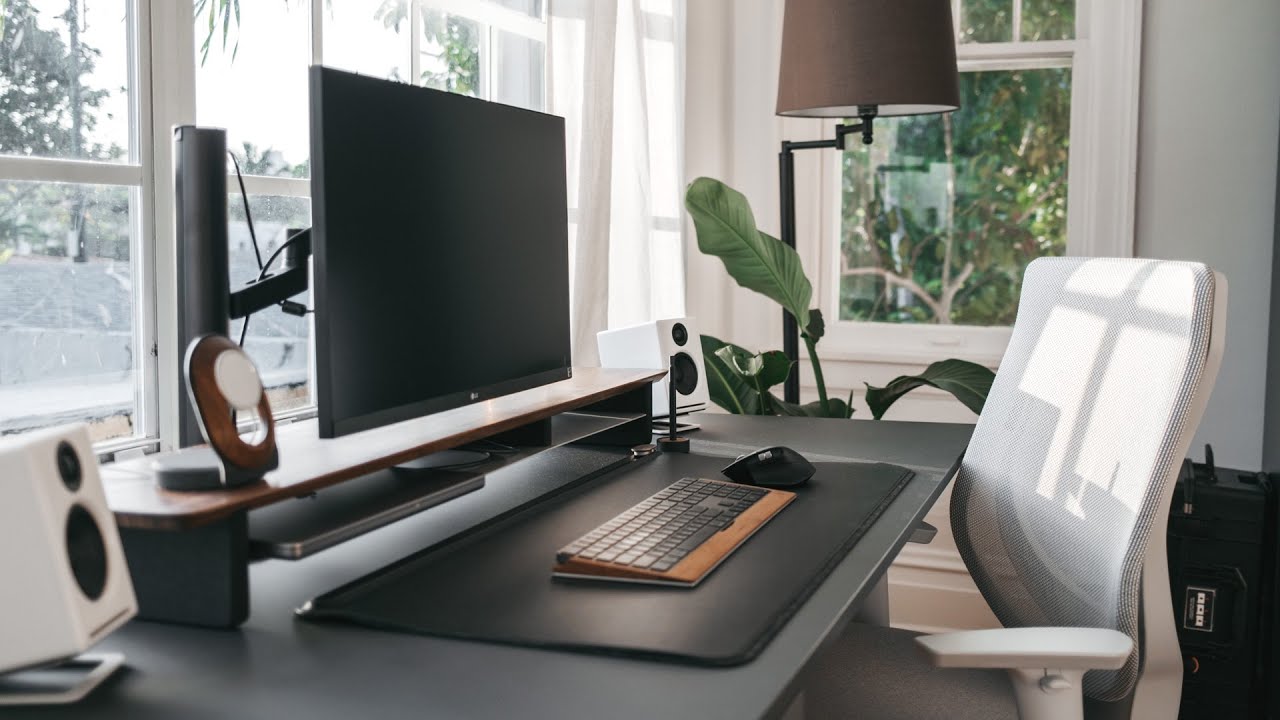The photograph showcases a meticulously arranged home office area. At the center is a gray desk, its surface largely occupied by a broad black mouse pad, a wood-grain keyboard with black keys, and a wireless black mouse. The desk features a small gray upright section at the back topped with dark wood, where an LG monitor is mounted on a versatile black swing arm. Flanking the monitor are white speakers with black faces. To the left of the setup, a white ergonomic office chair with gray mesh and white armrests stands ready. A fake indoor houseplant and a tall black lamp with a brown shade add homely touches to the scene. Large windows with white trim on gray walls let in sunlight, revealing a view of trees outside, enhancing the serene atmosphere of this functional workspace.